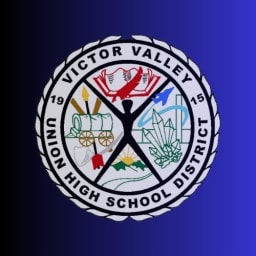This is an intricate logo for the Victor Valley Union High School District, established in 1915. The logo features a prominent circular design set against a background that shifts from dark navy blue on the left to a brighter royal blue on the right. Encircling the core of the logo, in black font, are the words "Victor Valley Union High School District" along with the founding year "1915."

Within the circle, a human-like figure with arms and legs outstretched, reminiscent of a stick figure, serves as the central element, dividing the logo into four distinct quadrants. Each quadrant contains a unique image: the top quadrant likely depicts a book, potentially with a red feather; the right quadrant features crystal-like structures with a jet flying around or emerging from them; the bottom quadrant showcases a rising sun over green mountains; and the left quadrant portrays a covered wagon pierced by a large arrow. This diverse imagery within the logo symbolizes the varied facets of the high school district's heritage and essence.